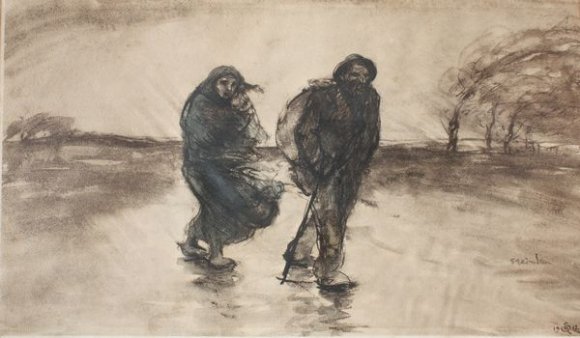The image is a detailed pencil drawing of an older man and woman walking through a violent storm. The scene is rendered with fast and loose sketches, primarily in muted shades of blue, black, gray, and white. The couple, depicted in 1800s-style attire, is at the center of the composition. The man, wearing a hat and a long jacket, carries a large pack on his back and a walking stick in one hand, while his other hand is in his pocket. The woman, adorned in a long, flowy dress, has a shawl or blanket draped over her shoulders, which flutters in the wind, along with her hair. The background features lightly sketched trees bending in the gale, reinforcing the severity of the storm. The ground beneath them appears to be a wet field, possibly with puddles, emphasizing the stormy conditions as they trudged together through the harsh weather.